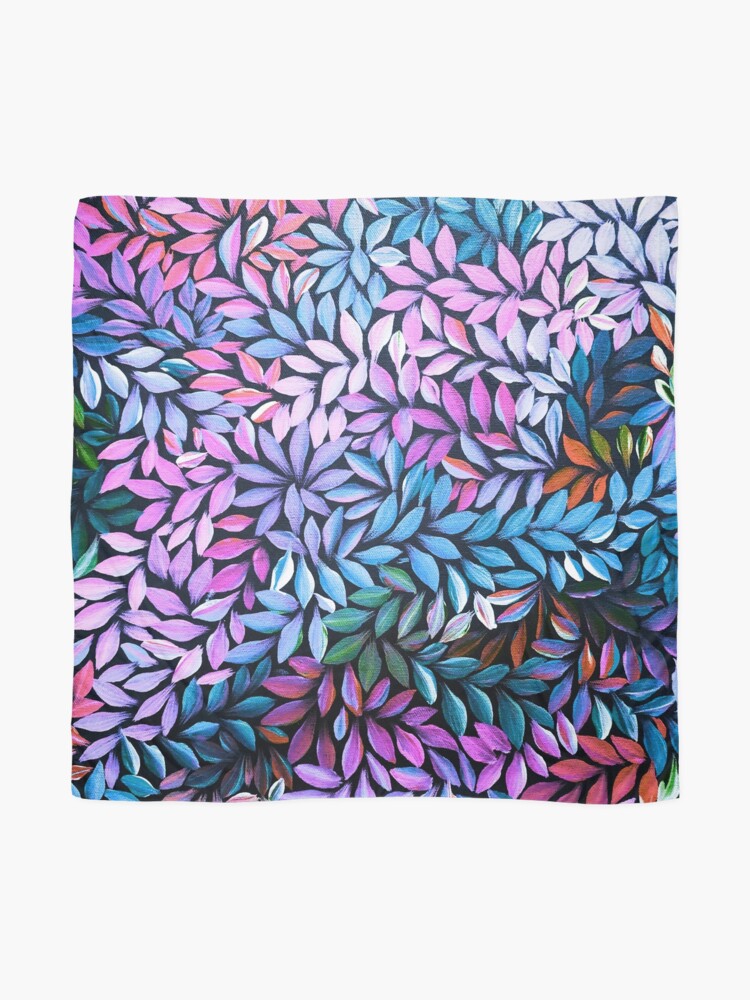A rectangular art print, approximately five to six inches in height and four inches in width, surrounded by a very light gray border. This border is about a quarter of an inch wide on the sides and an inch wide on the top and bottom, framing a central square that measures roughly two and a half inches on each side. This central square has wavy, irregular edges, resembling the texture of a piece of cloth, and is painted with an intricate floral pattern. The background appears black, enhancing the vibrant colors of various vine clusters and flowers that flow diagonally from the lower left to the upper right. The floral details include a mix of colors: greens, blues, purples, pinks, and reds. Specifically, the top left corner features pink flowers with hints of red and blue, transitioning into sections with light blue flowers, medium and dark blues, and various shades of purple, lilac, and pink. This pattern continues throughout, with clusters blending into each other, featuring occasional outlines and highlights in blue and green with some darker and lighter sections, creating a dynamic interplay of colors. The print showcases a mixture of floral elements with arrow-shaped leaves scattered throughout, creating an overall light and delicate appearance despite the complex and layered design.